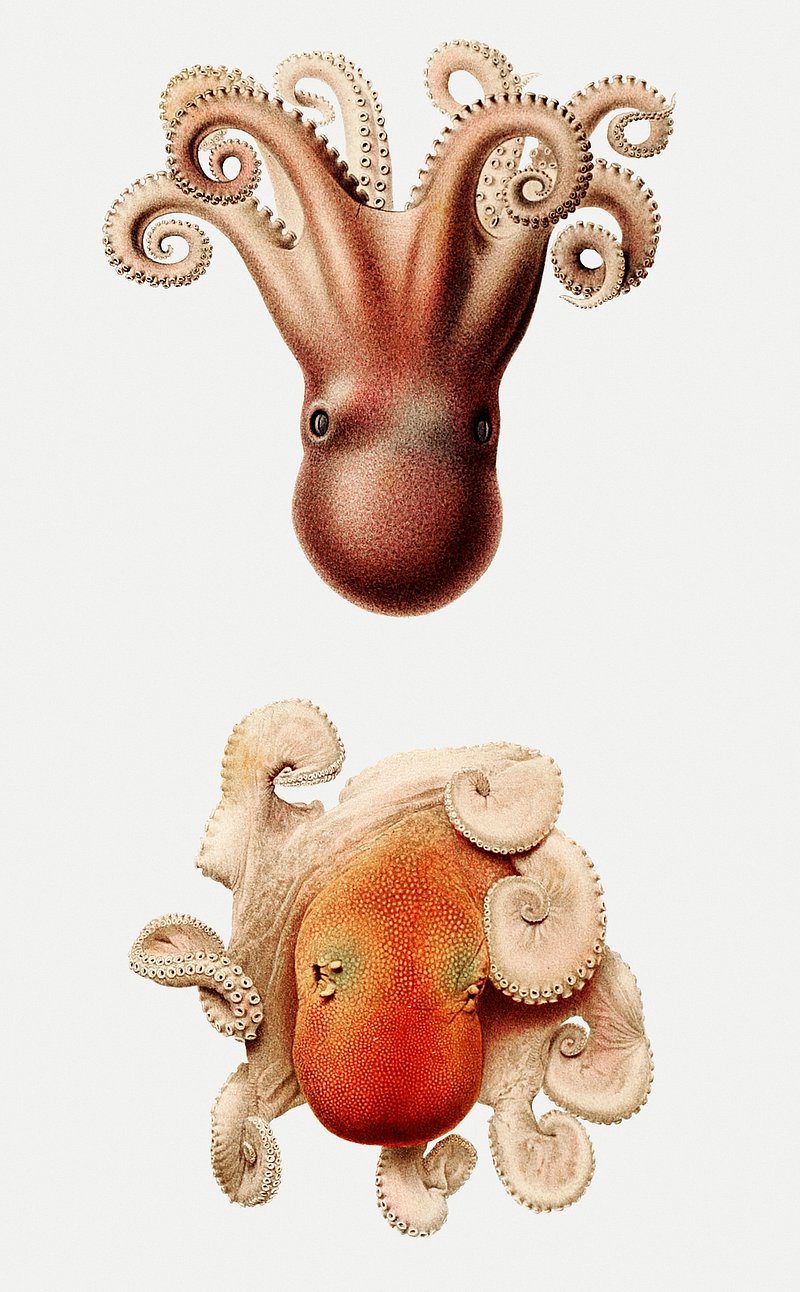This image features two octopuses positioned against a gray background, one placed above the other. The top octopus is depicted from a side view, showcasing a darker brown smooth outer skin with a slightly textured, speckled appearance. Its tentacles extend uniformly, revealing its suction cups. The tentacles have a gradient transitioning from dark brown to lighter shades of gray or pinkish tones. Its eyes are black and prominently visible. The bottom octopus is seen from a top-down view, highlighting its head and all eight tentacles. It has a distinct orange, pebbly-textured skin reminiscent of an orange peel, with tentacles that are light gray or white, sprawled out in various directions, giving it a scrunched, more dynamic appearance. Both octopuses, though different in color and texture, exhibit realistic, lifelike details, suggesting a high level of artistic or photographic realism.